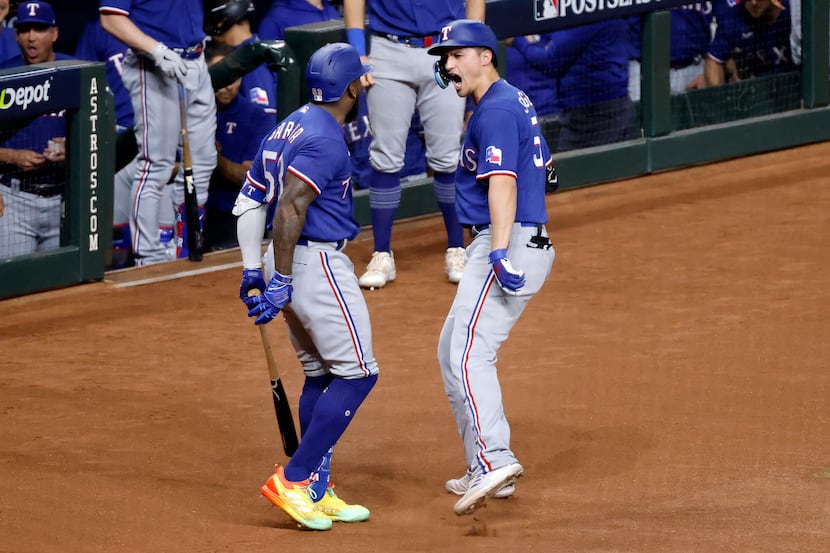This image captures an intense moment at a baseball game with two players from the Astros team's minor league, both wearing bright blue jerseys and gray pants with a red, white, and blue stripe down the side. The player on the left, an African American man with a short beard, is seen leaping off the ground, wearing knee-high blue socks and vibrantly colored cleats that fade from yellow to orange to green. He holds a bat with both hands behind his back. The player on the right, a white man with short, trimmed light hair, is also in mid-air, wearing white cleats and a glove on his left hand. Both players are wearing blue helmets and are caught in a moment of passionate hype or perhaps confrontation, seemingly shouting at each other. Behind them, a grid-like fence with a puffy green border surrounds the dugout, where other team members in identical uniforms are lined up. The fence carries the "astros.com" branding, adding to the vibrant atmosphere of the game.